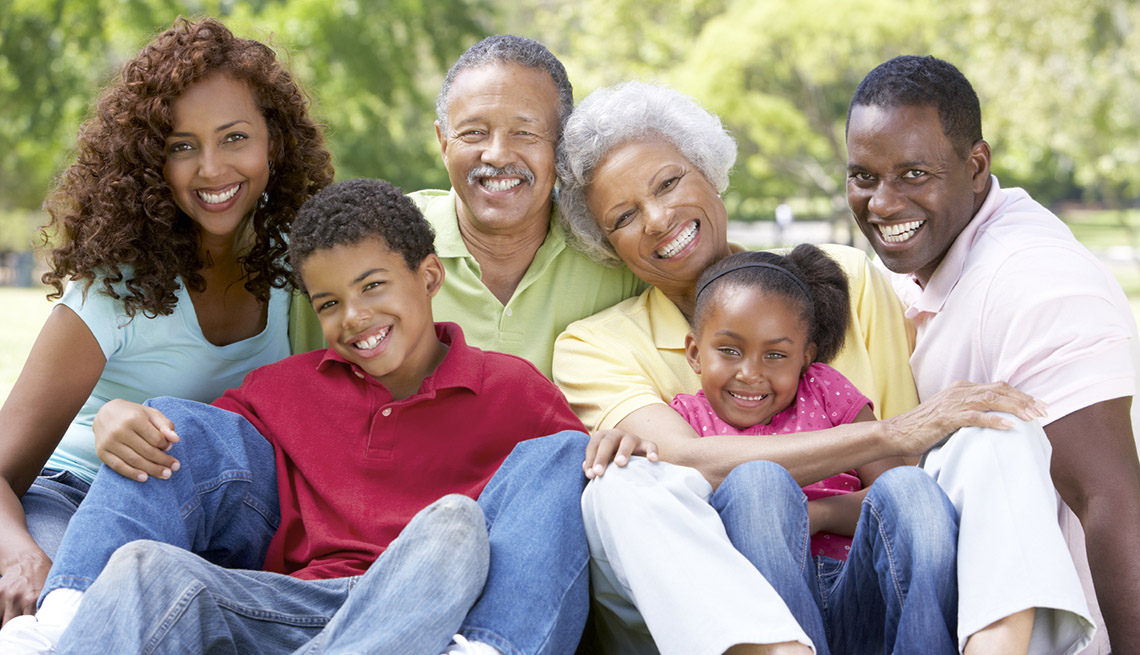In this vibrant and heartwarming photograph, a joyful African-American family is gathered together on a bright summer day, seated on the ground with a backdrop of blurred greenery that suggests they are in a park. Starting from the right, there is a smiling man in his 30s or 40s, wearing a light pink polo shirt and sporting short black curly hair. Beside him, an elderly grandmother with white curly hair, dressed in a yellow polo shirt and white pants, embraces a young girl around eight years old, who has her hair in a ponytail with a headband and light eyes, and is wearing a pink t-shirt. The grandmother leans her head on the shoulder of her husband, an elderly man with salt-and-pepper hair and a mustache, clad in a green polo shirt. In his lap sits a 12-year-old boy with short curly hair and a red polo shirt, leaning back comfortably against his grandfather. To the far left is the mother, a woman with beautiful brown curly medium-length hair and a radiant smile, dressed in a light blue top paired with denim. The family is collectively exuding happiness and unity, making for a picture-perfect moment.